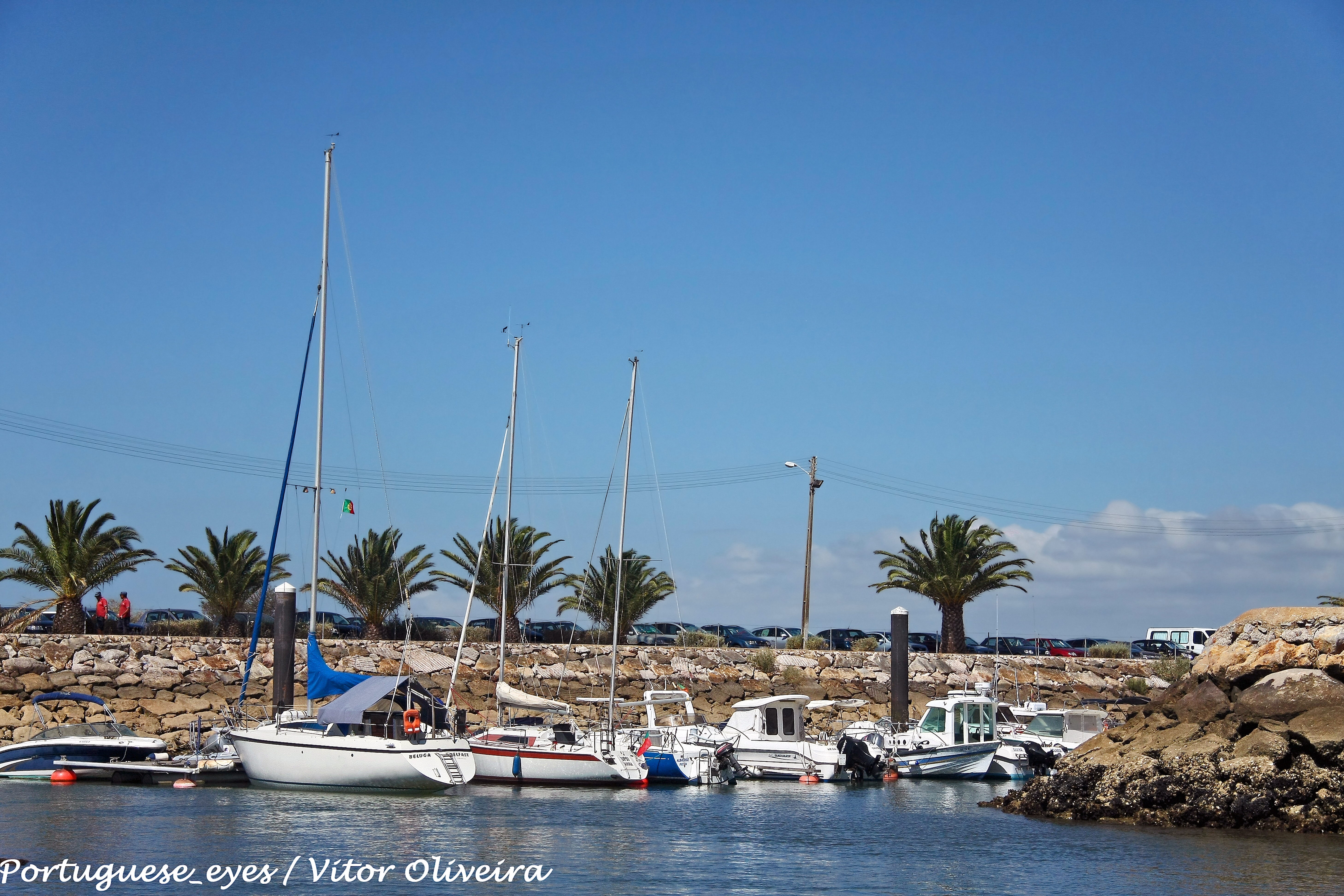This photo captures a serene seaside scene with a variety of boats docked in calm, blue waters. In the center of the image, three sailboats with visible but unraised masts are prominently featured among other powerboats. The boats, approximately eight to ten in number, are stationary, indicating a peaceful marina. To the right, the water is bordered by rock walls, and in the background, a parking lot with parked cars and several people is visible. Palm trees add a tropical touch to the landscape. The sky, occupying the top two-thirds of the image, is adorned with scattered clouds. In the bottom left-hand corner, white text reads "Portuguese_eyes / Vitor Oliveira," crediting the photographer.